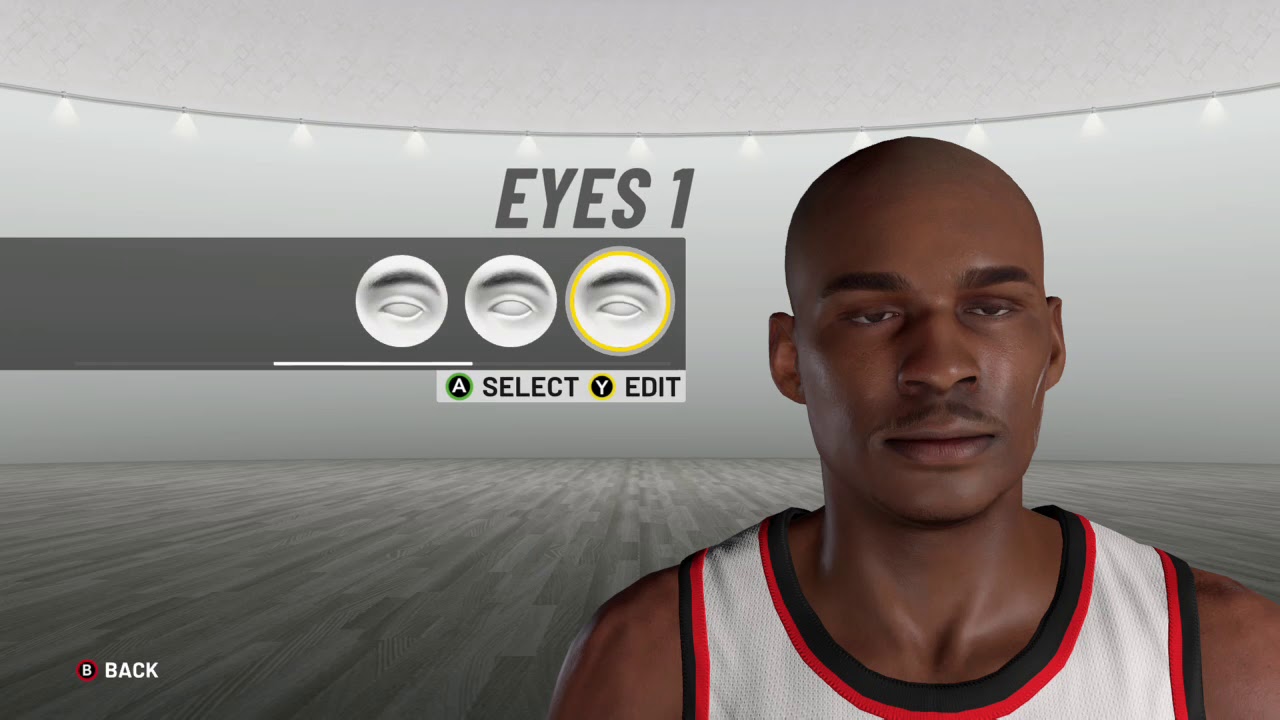The image portrays a digitally created African-American basketball player, prominently positioned to the right of the frame. He appears to be in his late 20s, with a shaved head, shaded mustache, and brown eyes. He is dressed in a white jersey accented with blue and red stripes along the sleeves and neckline. 

In the background, the scene is set in a large basketball court or arena rendered entirely in shades of gray. The expansive court is open and features a gray wall with 14 evenly spaced lights along the seam where the wall meets the ceiling, which is also gray.

To the left of the basketball player in the foreground, there is a graphic element labeled "Eyes 1" in a gray font, approximately 12 to 14 points in size. This graphic includes a selection box displaying three eyes with an eyebrow above each, indicating a focus on eye selection. At the bottom of this selection box, there are two smaller boxes: one green labeled "Select" and the other yellow labeled "Edit."

In the bottom left corner of the image, there is a white letter "B" within a red circle, resembling a button, with the word "back" next to it, suggesting that clicking this area would navigate back to a previous screen or interface. 

Overall, the image combines elements of AI-generated art and interactive design, situated within a monochrome depiction of a basketball stadium.